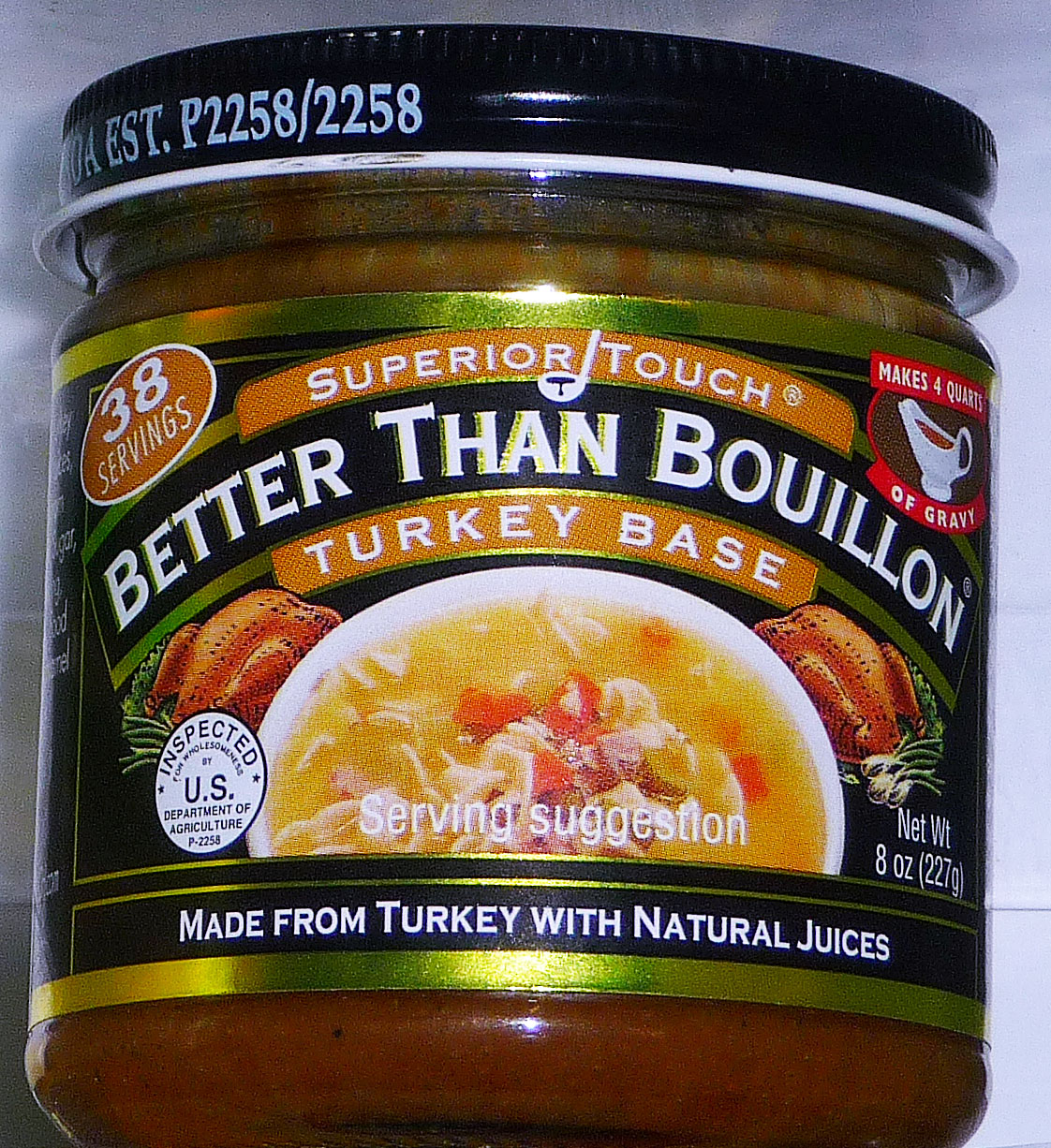This close-up image features a food product packaged in a glass bottle. The bottle is topped with a black lid adorned with white lettering, which reads "EST. P2258." Inside, the bottle contains a vibrant red substance. The label, centered prominently on the bottle, showcases a bowl of soup that closely resembles chicken noodle soup. The soup appears yellow, served in a white bowl, and includes visible pieces of meat and carrots. The label is branded with the name "Superior Touch" and provides product details including "38 servings," and "Makes four quarts of gravy." It specifies that the product is "Better Than Bouillon, Turkey Base," highlighting that it is "Made from turkey with natural juices." The net weight of the contents is listed as 8 ounces.